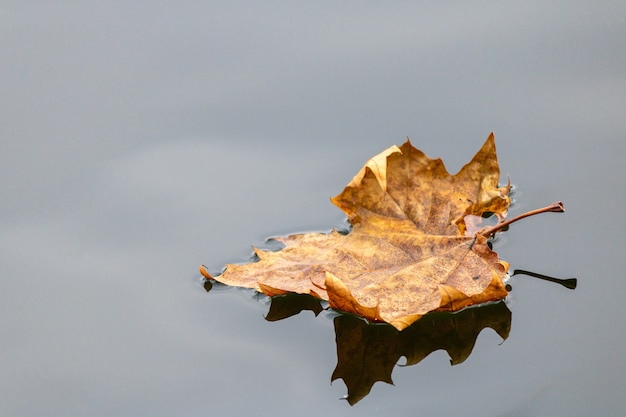The photograph captures a dried, yellowish-brown leaf floating on an almost motionless body of water. The leaf, the image's focal point, appears to be face down, displaying its intricate veins and serrated edges. Positioned slightly toward the right, the leaf is slightly crumpled and shows signs of age and decay. The calm water reflects the leaf and hints of a cloudy sky, creating a serene yet somber ambiance. The light gray water, with subtle cloud reflections, enhances the leaf's autumnal orange and amber tones. The scene suggests a quiet moment, perhaps in a lake or a still puddle, with a faint water tension around the leaf emphasizing its delicate, floating state.